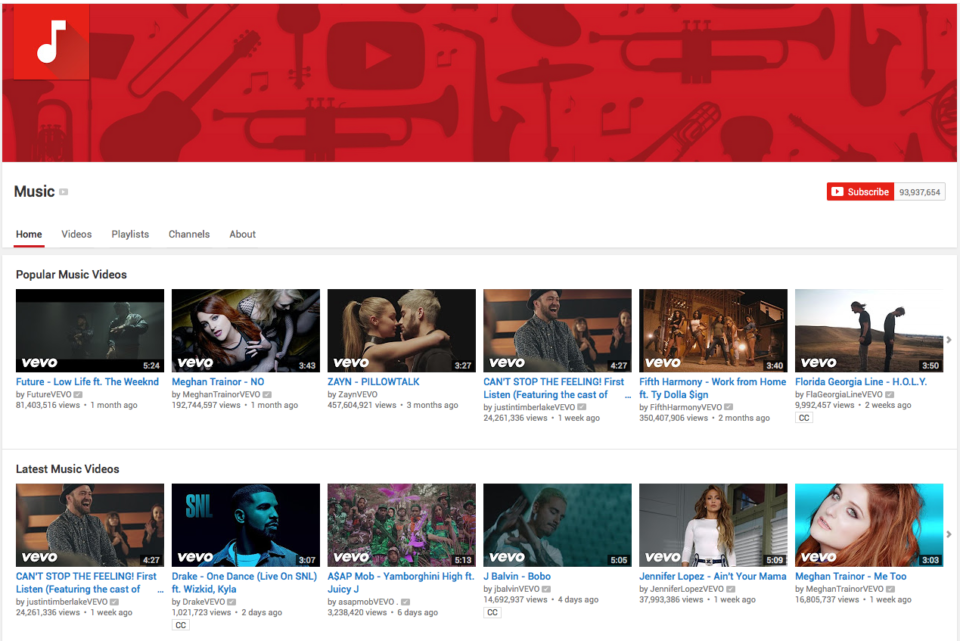This screenshot captures the YouTube Music channel page, currently displaying the homepage. The banner showcases a vibrant red graphic featuring the YouTube logo surrounded by various musical instruments, predominantly brass, along with musical notes. Specific instruments visible include guitars, trumpets, tubas, saxophones, and clarinets.

The title of the channel is simply "Music." Directly beneath the banner, on the right, is a prominent red subscribe button, indicating that the channel boasts 93,937,654 subscribers. There are five navigational tabs available: Home, Videos, Playlists, Channels, and About, with the Home tab currently selected.

In the Home section, a playlist titled "Popular Music Videos" is prominently displayed, featuring six music videos. Another playlist, named "Latest Music Videos," is positioned below the first, also containing six videos from a variety of artists. Both playlists are arranged horizontally, showcasing the most recent uploads ranging from two days to two months old at the time the screenshot was taken.